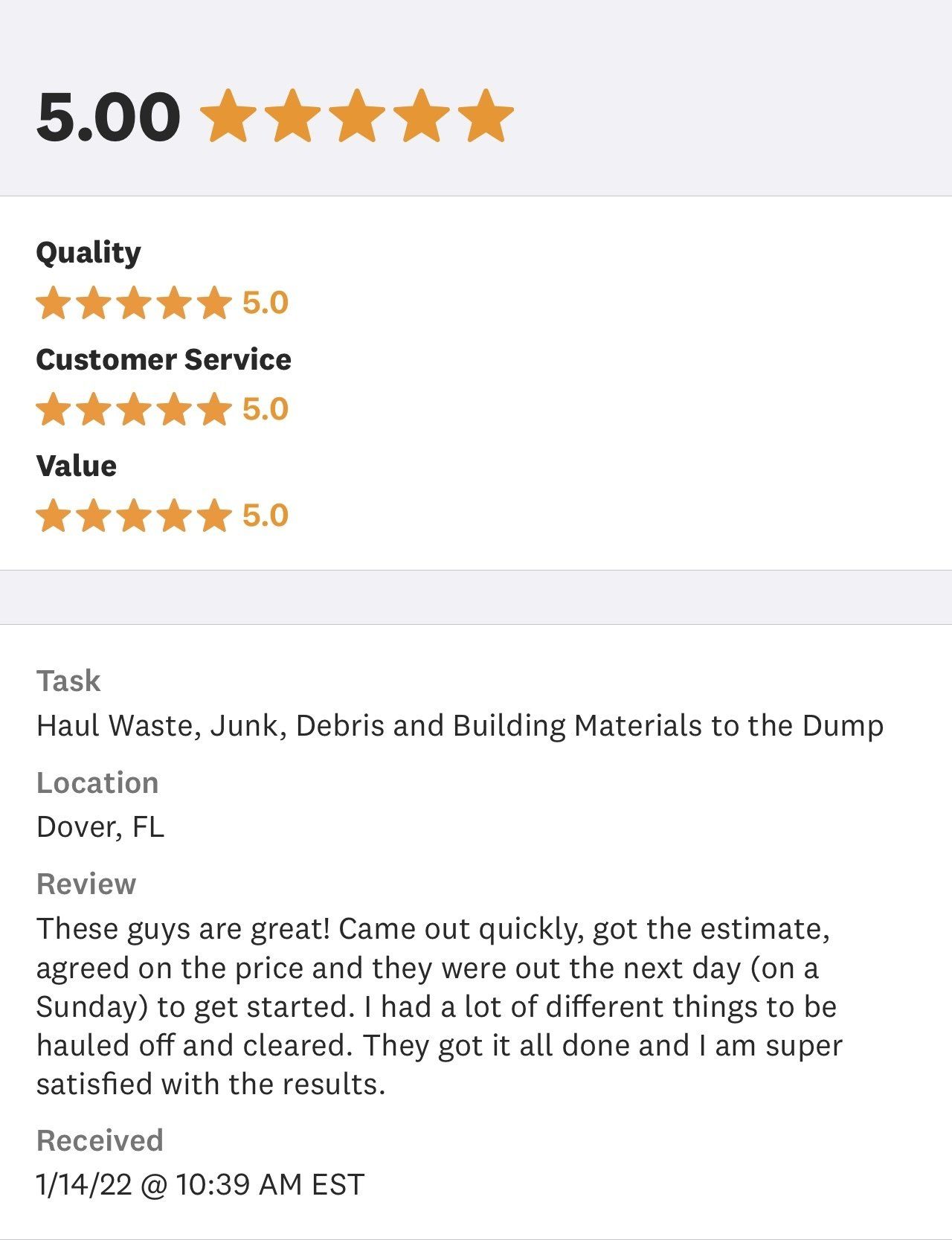**Rating Summary**

At the top, a large grey box prominently displays the rating. To the left, the rating shows "5.00" in bold black text. Inside the box, there are five filled stars with small orange stars below, signifying the highest rating.

The detailed breakdown includes:
- **Quality:** Indicated with five stars and "5.0" in yellow text.
- **Customer Service:** Also represented with five stars and "5.0" beneath it in black text.
- **Value:** Displayed with five stars and "5.0" below.

Underneath this rating box, another grey bar separates the sections.

The text below provides more specific details:
- **Task:** In dark grey text, followed by "Hallways, junk, debris, building materials to the dump" in black text.
- **Location:** In dark grey text, with "Dover, Florida" in black text below.
- **Review:** In dark grey text, followed by the review in black text: "These guys are great! Came out quickly, got the estimate, agreed on the price, and they went out the next day on a Sunday to get started. I had a lot of different things to be hauled off and cleared. We got it all done, and I'm super satisfied with the results."

The final line indicates the receipt of the service:
- **Date and Time:** "1-14-22 at 10:39 AM EST" in dark grey text.